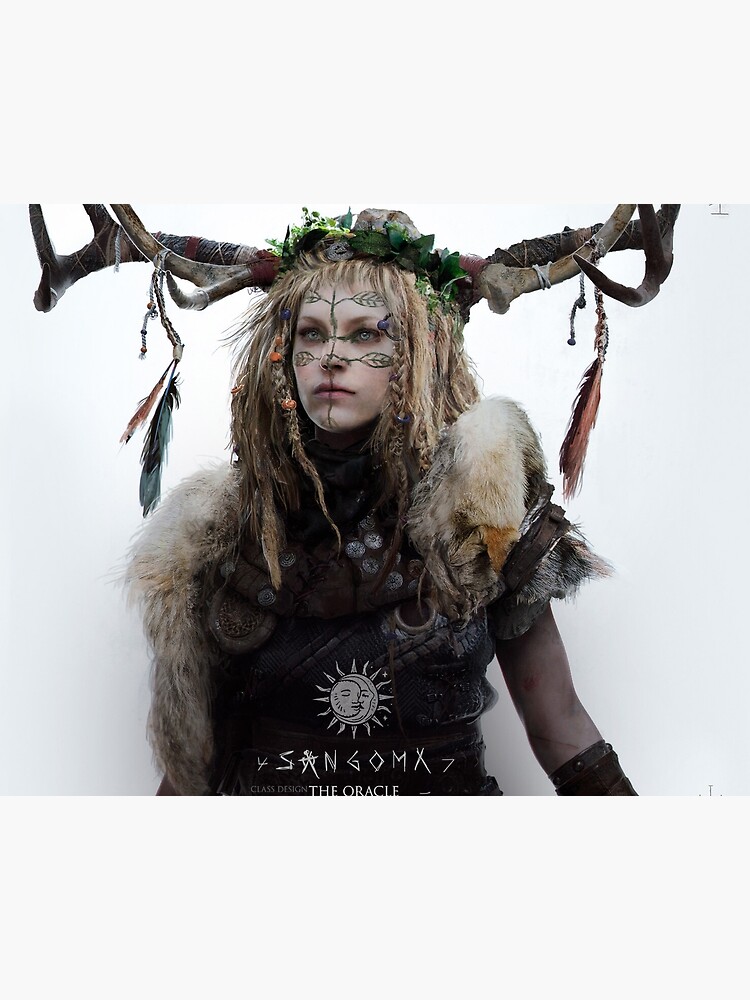This image features a captivating woman in the center, designed to evoke a fantasy or mystical theme reminiscent of ancient times, possibly inspired by Vikings or a fantasy show. She has striking blonde hair styled in dreadlocks and braids, adorned with beads. Atop her head, she wears an elaborate headpiece resembling antlers made of wood, adorned with a wreath of green leaves. Various feathers hang from the antlers, including a green feather on the left, a smaller orange feather above it, and a reddish-brown feather on the right.

Her face is painted with intricate designs of leaves and lines in green, extending across her cheeks, forehead, and down to her chin, enhancing her otherworldly appearance. She wears a black shirt under a voluminous fur cape that transitions from white at the shoulders to a darker, blackish hue further down. Below her, the image bears the symbols of the sun and moon in white, followed by the text "Sangoma" and "the Oracle," signifying her mystical role.